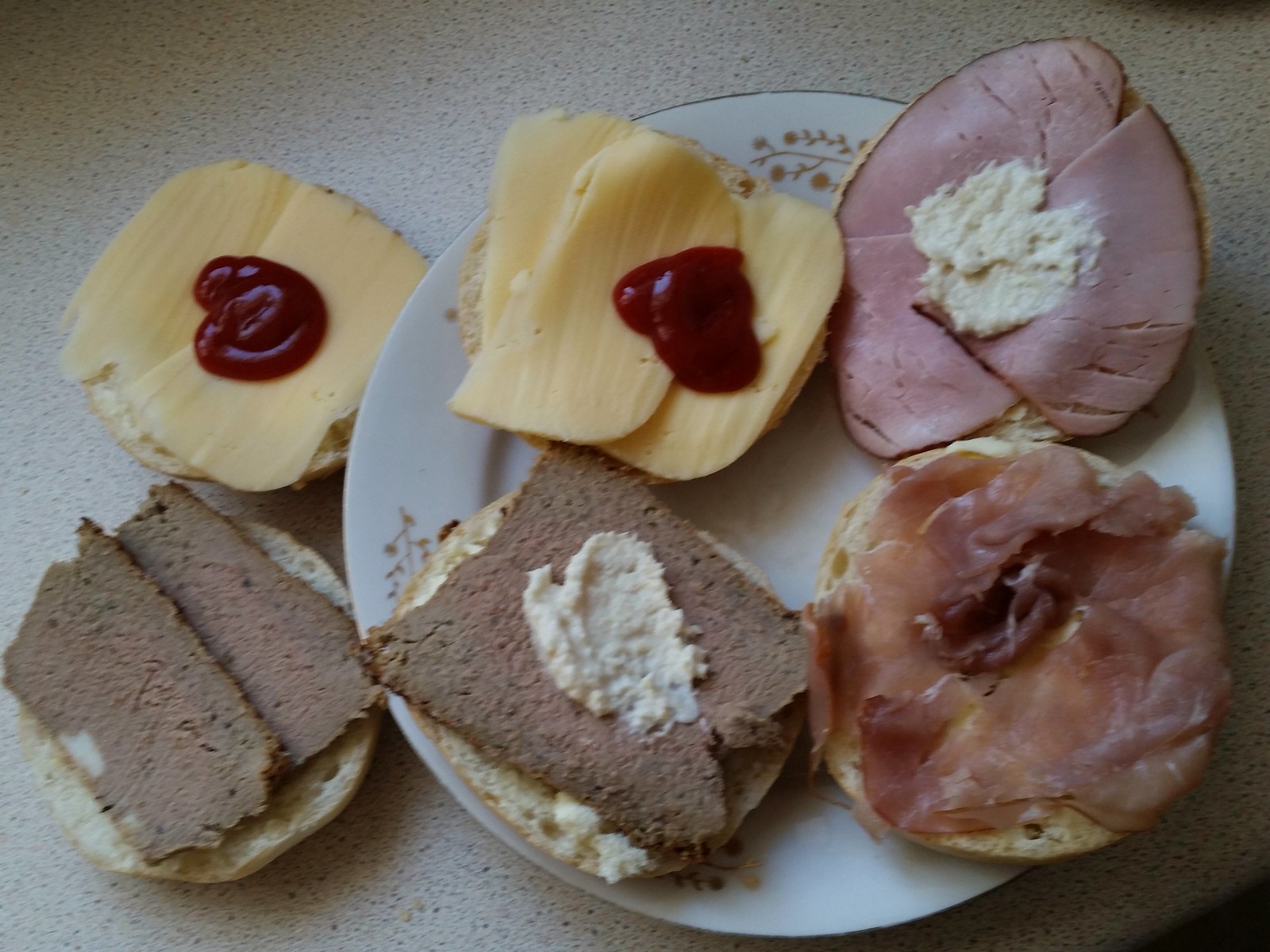This indoor photograph shows a meticulously arranged display of open-faced sandwiches, captured from a top-down perspective on a light gray granite countertop with dark gray and black flecks. The sandwiches are presented on a white porcelain plate adorned with a brownish floral design along the rim. 

There are six individual slices of bread, each topped with various ingredients. On the top left, a sandwich features a slice of bread with cheese and a dollop of ketchup. Directly next to it, another bread slice is topped with cheese and roast beef, finished with a similar ketchup or marmalade topping. The third sandwich includes bread topped with a piece of meat, which appears to be prosciutto, and is layered with cream cheese. 

Moving to the bottom row, the first sandwich showcases a round piece of bread with bacon, while the sandwich to its right features what looks like ham spread with cream cheese. The final bread slice on the bottom right is topped with meat and a generous layer of cottage cheese. The arrangement is slightly asymmetrical, with two of the sandwiches placed off to the side of the central plate, adding an artisanal touch to the visually appealing presentation.